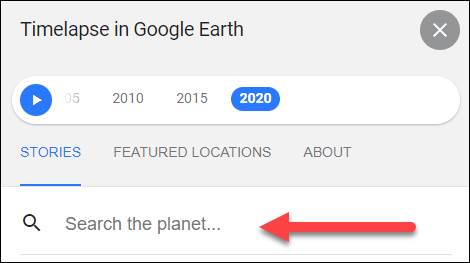The image features a simplistic design set against a gray and white background. Encased in a thin black-lined rectangular border, the scene is focused primarily on a prominent search bar. Located in the bottom left corner, a magnifying glass icon symbolizes the search function. To its right, the phrase "Search the planet..." prompts user interaction.

A large, photoshopped red arrow, complete with a subtle gray shadow, points leftward towards the search bar, emphasizing its importance. In the upper right-hand corner, a gray circle with a white 'X' serves as a close button for the tab.

The header contains the text "Time-lapse in Google Earth" in bold black font, positioned in the upper left corner. Just below, a white bar displays a blue circle with a white play button and the numbers "05", "2010", "2015", and "2020." The year "2020" is highlighted in white font within a blue circle, indicating it is currently selected.

Further down, navigation options list "Stories," "Featured Locations," and "About." "Stories" is highlighted with blue text and an underline, marking it as the active section. Overall, the image visually guides users towards exploring time-lapse features in Google Earth, utilizing clear indicators and highlighted elements.